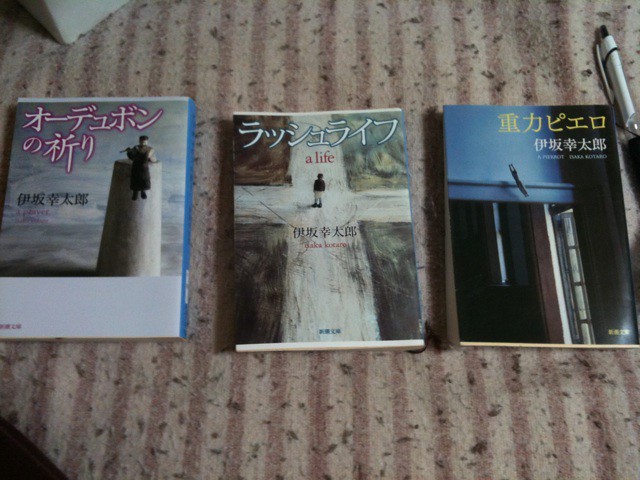This image features three distinct Asian booklets displayed on a table with a pink and off-white striped tablecloth featuring green specks. From left to right, the booklets differ in their cover designs and features. The left booklet showcases a person at the top of what appears to be a tower or silo, set against a blue sky with white clouds. It has white Asian characters trimmed in red along the top edge. The middle booklet depicts a person standing at a crossroads, characterized by a large cross-like intersection on a dirt road. This cover is predominantly blue with white Asian writing at the top, red text reading "A Life" below it, and additional red and black Asian characters at the bottom. The right booklet, which lacks any human figures, appears to feature a darkened window or entrance with both yellow and white Asian characters on the cover. Completing the scene, a silver pen with a black tip is positioned at the upper right corner, partially intruding into the frame from the right.